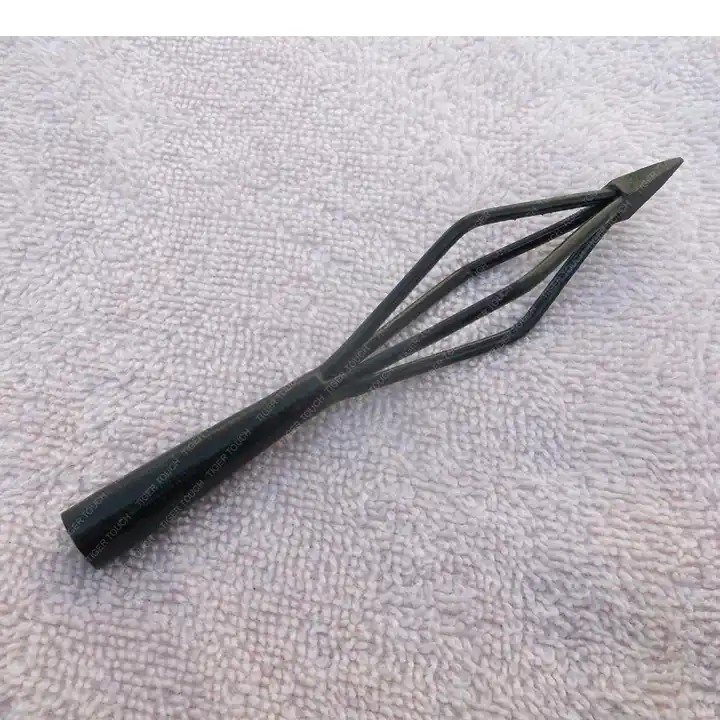The image showcases a unique, black metal contraption with a sharp, pointy tip at one end. The object is composed of four protruding, angled mini poles that connect the pointed end to a handle. The metal appears slightly worn and not a pure black, indicating some use or age. The contraption, whose shape resembles an old-fashioned whisk or even a lava lamp, sits atop a fabric surface that seems to be a white towel or carpet, distinguishing itself from the textured background. Notably, the handle is inscribed with the name "Tiger Touch," providing a clue, yet no concrete understanding of its specific purpose or origin. The image itself bears a watermark with the same "Tiger Touch" inscription multiple times, centered neatly within the frame.